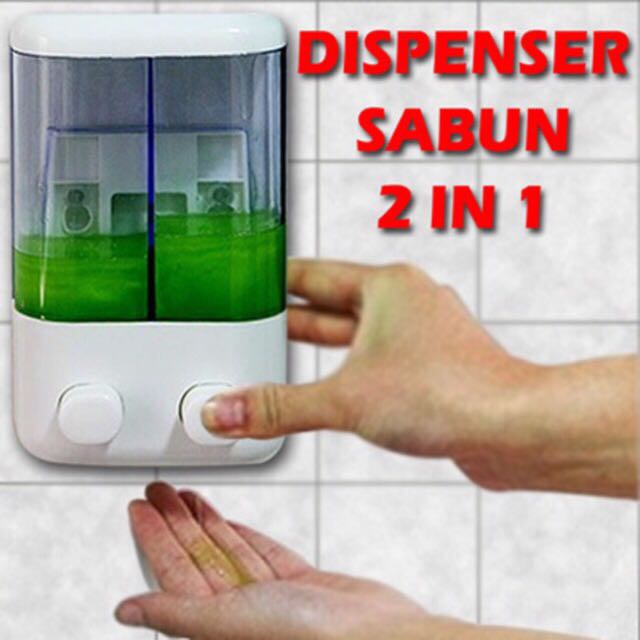The image portrays a white, dual-compartment soap dispenser with clear plastic chambers mounted against a bathroom-tiled wall. Each chamber contains a green liquid soap, with the right chamber visibly more filled than the left. In the image, a right hand is pressing the chunky plastic button on the right chamber, dispensing soap into the left hand below. The text "DISPENSER SABUN 2-IN-1" appears in bold, red uppercase letters with a drop shadow, positioned in the upper right corner of the image. The soap dispenser features a white top and bottom, and the setting suggests it's inside a bathroom, although there is speculation it might have been photoshopped due to the visible fingers behind the dispenser. The overall image is perfectly square in nature and appears to be a low-resolution advertisement.